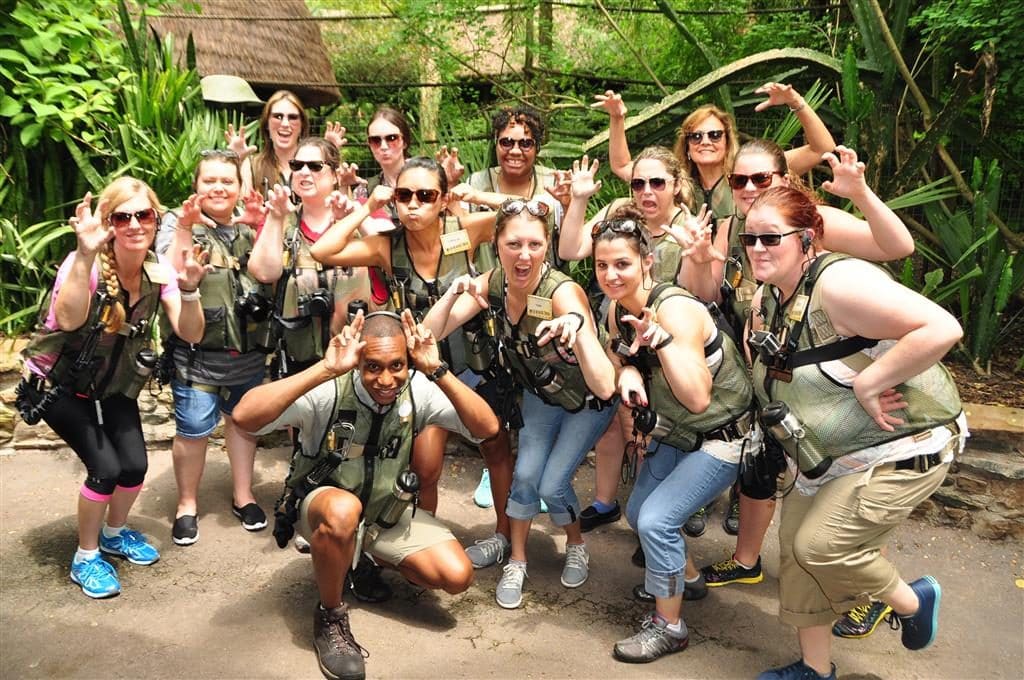In an outdoor setting reminiscent of a jungle atmosphere, a large group of women—primarily Caucasian with a couple of women of color—pose joyously in front of a hut's roof barely visible in the background. The women, wearing an assortment of blue jeans, khakis, and leggings, are dressed in green sleeveless vests with sleeveless tops, hinting at warmer weather. Most of them sport dark sunglasses and appear sweaty and somewhat tired, possibly from a recent accomplishment. Many have water bottles strapped to their vests. In the midst of the group, an African-American male squats with hands positioned like ears on either side of his head, while the women around him strike playful claw-like poses. The group is gathered on what seems to be a concrete road, with a retaining wall and lush vegetation encompassing trees and various plants behind them, enhancing the lively and animated feel of the scene.